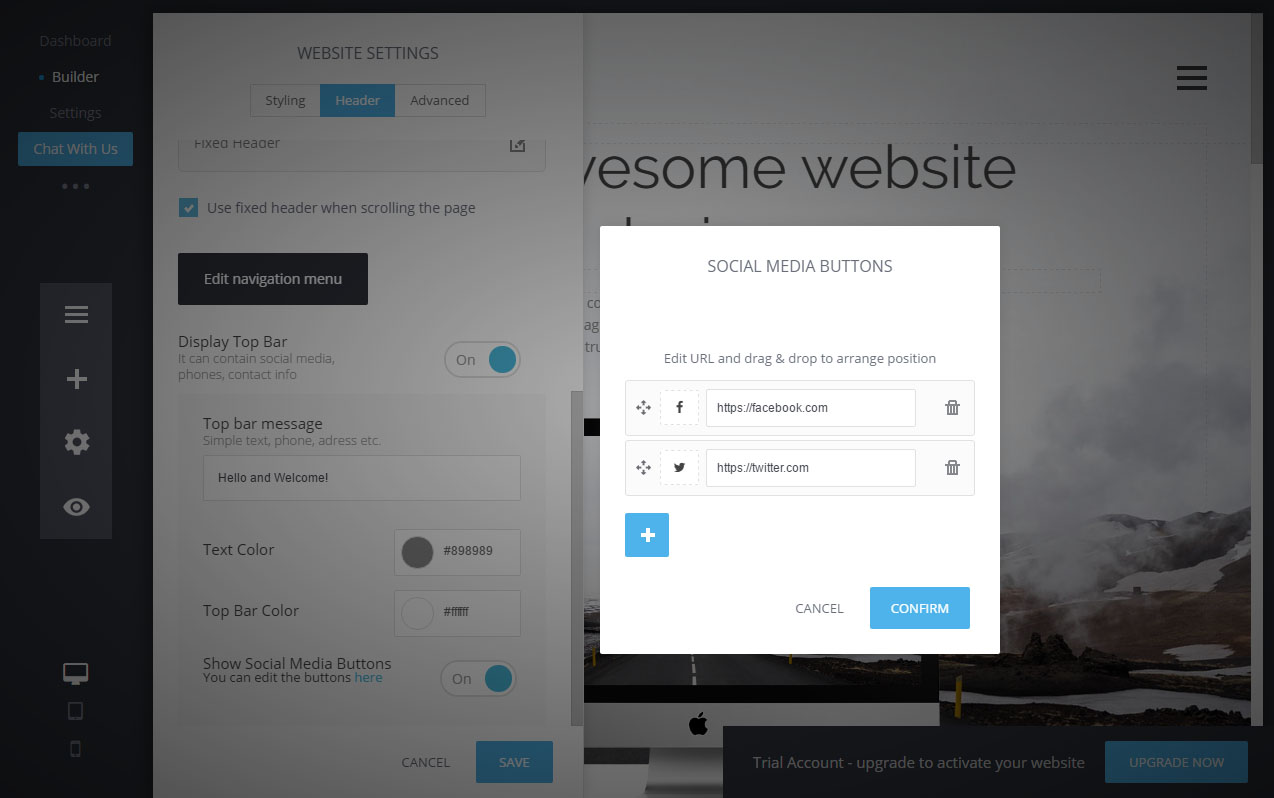The image showcases a website builder interface. On the left side, a vertical black toolbar features various tabs such as "Builder" and "Chat with Us," along with a menu button, a plus button, a settings gear icon, and an eyeball icon for previewing. At the bottom of this toolbar are icons representing different device views: a desktop PC, a tablet, and a mobile device.

To the right of the toolbar is a white window labeled "Website Settings," offering various options for customization and configuration of the website. Further right, the main workspace displays a cloudy mountain background, presumably the landing page of the site being built. In the foreground, a white pop-up window labeled "Social Media Buttons" allows the user to add buttons for various social media platforms.